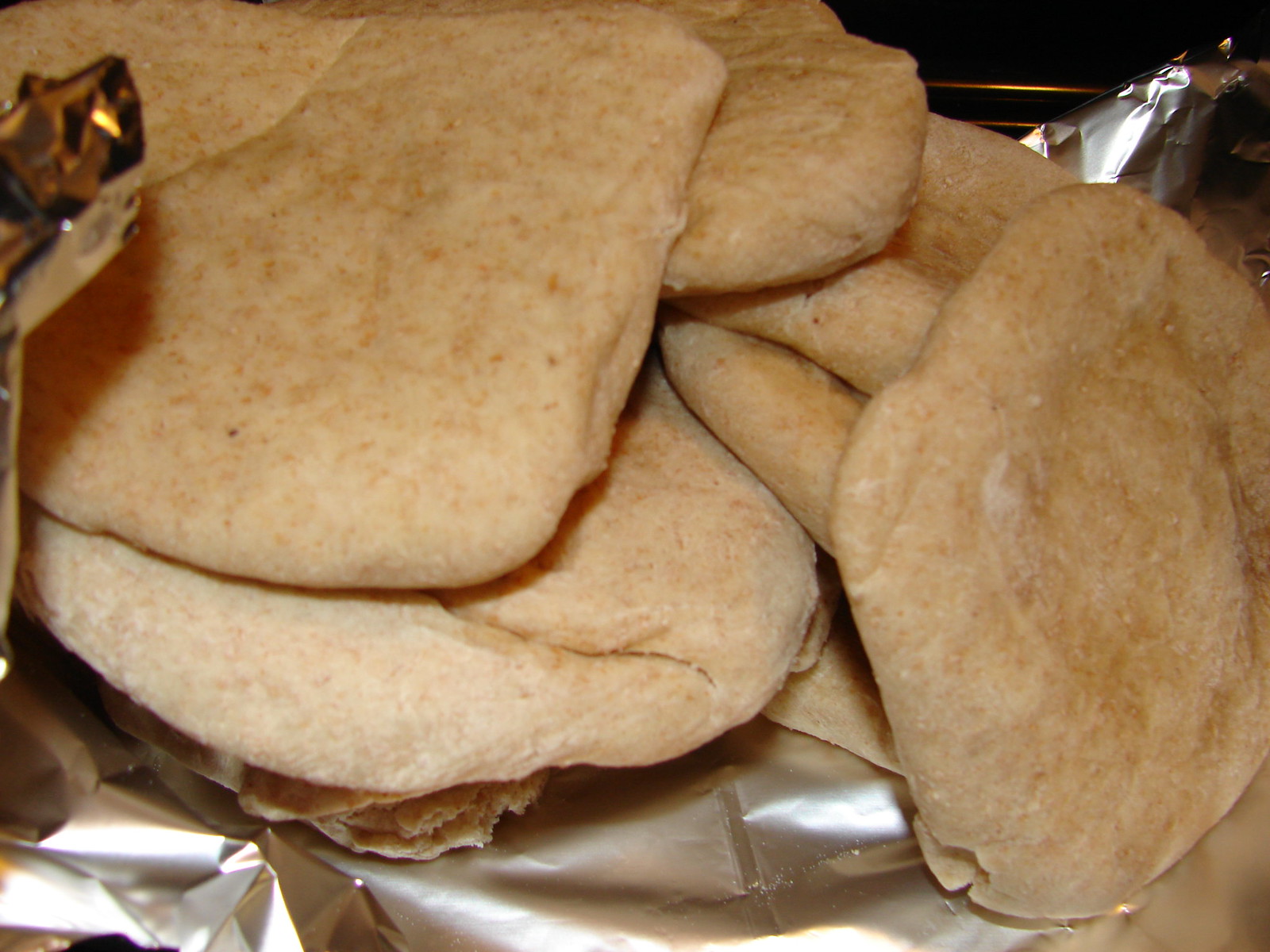In this detailed, zoomed-in photo, we see a shiny steel aluminum foil tray filled with numerous baked bread items that resemble flour tortillas or cookies. The food is characterized by its yellow-white color with dark brown speckles, giving an impression of slight crispiness while also appearing soft. They are stacked in a disorderly fashion, some overlapping and piled on top of each other, totaling around 15 to 20 pieces. One of the pieces at the bottom appears slightly ripped, revealing a fluffy, white, and somewhat crumbly interior. The bread pieces are mostly rectangular with curved edges. The aluminum foil, slightly bent and stretched, is holding the bread items in place within the tray. In the background of the photo, there is a stark contrast provided by a dark wall or unlit area, emphasizing the focus on the bread and foil.